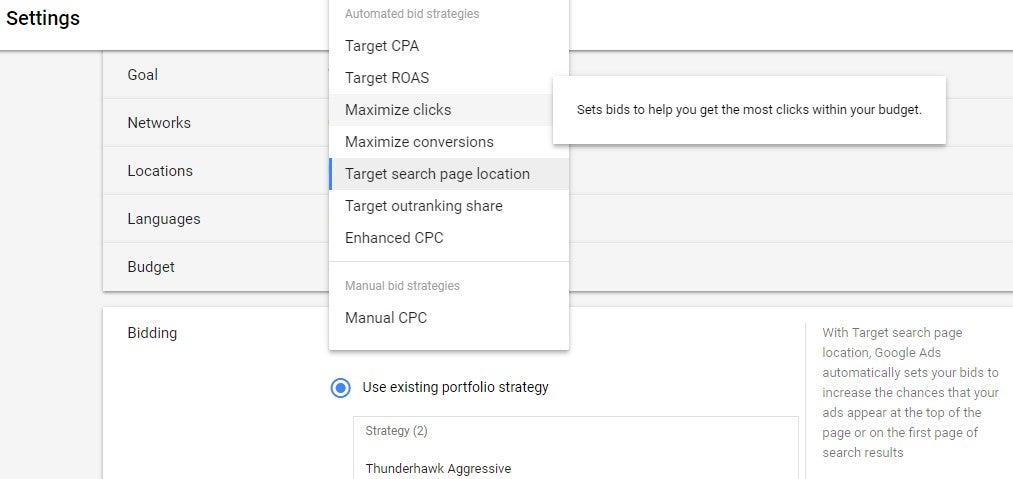Screenshot of Google Ads Settings Page:**
  
The image is a detailed screenshot taken from a computer displaying the Google Ads settings interface. At the top left, the header clearly shows the word "Settings." Below this header, there are several dropdown arrows corresponding to different configuration categories including "Goal," "Networks," "Locations," "Languages," and "Budget."

In the center of the screenshot, a pop-up window titled "Automated Bid Strategies" lists various bidding options. These include:

- Target CPA
- Target ROAS
- Maximize Clicks (highlighted)
- Maximize Conversions
- Target Search Page Location
- Target Outranking Share
- Enhanced CPC

Following this, the screen displays "Manual Bid Strategies" which include "Manual CPC" among other options. 

Highlighted with a blue circle, the phrase "Exist a Portfolio Strategy," along with "Strategy Two," and "Thunderhawk Aggressive," suggests an advanced, customized approach to bidding.

In a separate box on the bottom right, the text explains the function of the "Target Search Page Location" strategy: "With Target Search Page Location, Google Ads automatically sets your bids to increase the chances that your ads appear at the top of the page or on the first page of search results."

Overall, this screenshot captures the detailed settings page of a Google Ads account, likely belonging to an individual fine-tuning their advertisement campaign to ensure optimal visibility and performance.